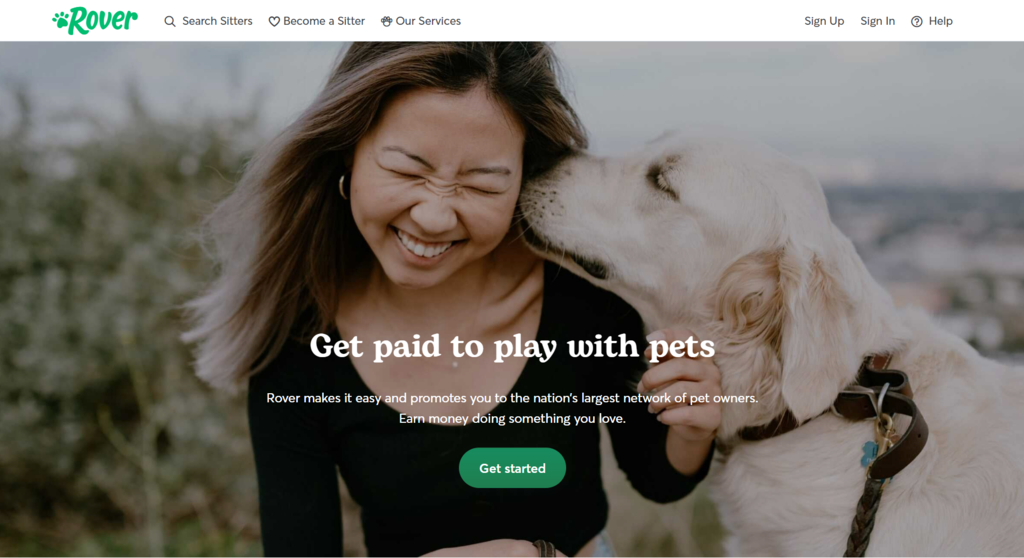Sure, here is a cleaned-up and detailed caption:

---

This screenshot captures the homepage of the Rover website, distinguished by its green theme. In the top left corner, the Rover logo features the brand name "Rover" in green next to a green paw print. Immediately to the right of the logo are three navigational options: "Search Sitters" accompanied by a magnifying glass icon, "Become a Sitter" with a heart icon, and "Our Services" with another paw print icon. To the far right of the same navigation bar are links for "Sign Up," "Sign In," and "Help."

The background of the webpage showcases a heartwarming image of a joyous woman in her 30s being affectionately kissed on the face by a golden retriever. Overlaid on this picture is a prominent white text that reads, "Get paid to play with pets." Below this, in smaller white text, it explains, "Rover makes it easy to connect you to the nation’s largest network of pet owners. Earn money doing something you love." At the bottom of the image, there's a green button labeled "Get Started."

---